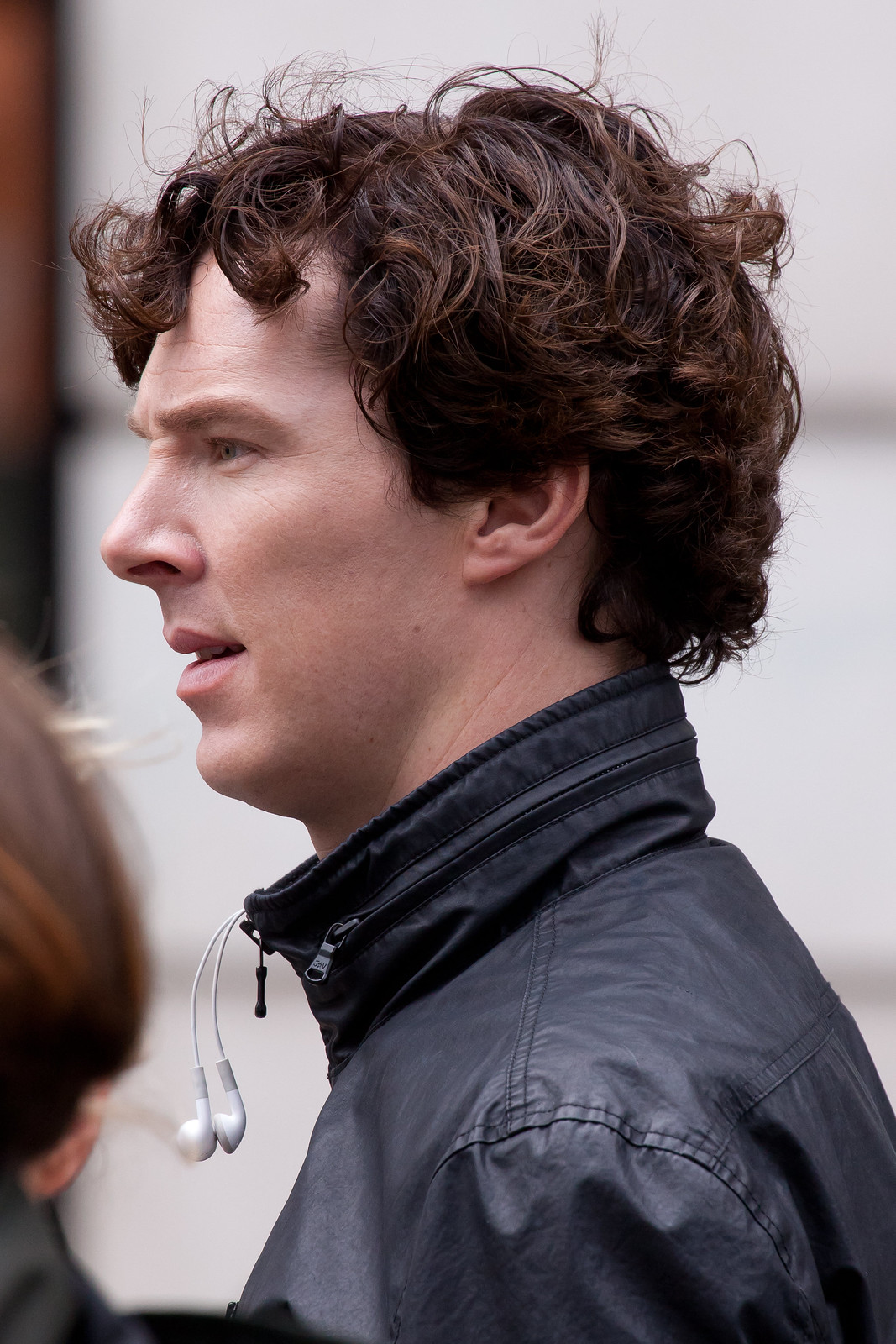In the image, a young man with dark, wavy hair is the central focus. He is wearing a black leather jacket with a noticeable zipper near the top and has small in-ear earphones hanging from his jacket. The man's mouth is slightly open as he looks intently to the left side of the image, his expression suggesting deep thought or focus. The background of the image is mostly blurred, appearing to be either the side of a wall or a building, set against a very light, almost white backdrop, giving the impression of an outdoor setting in the middle of the day. The wind seems to be gently blowing his hair. In the bottom left corner, a partial head is visible, cut off and out of focus, adding an extra layer of depth to the image. The overall color palette includes shades of black, white, gray, brown, tan, and off-white.